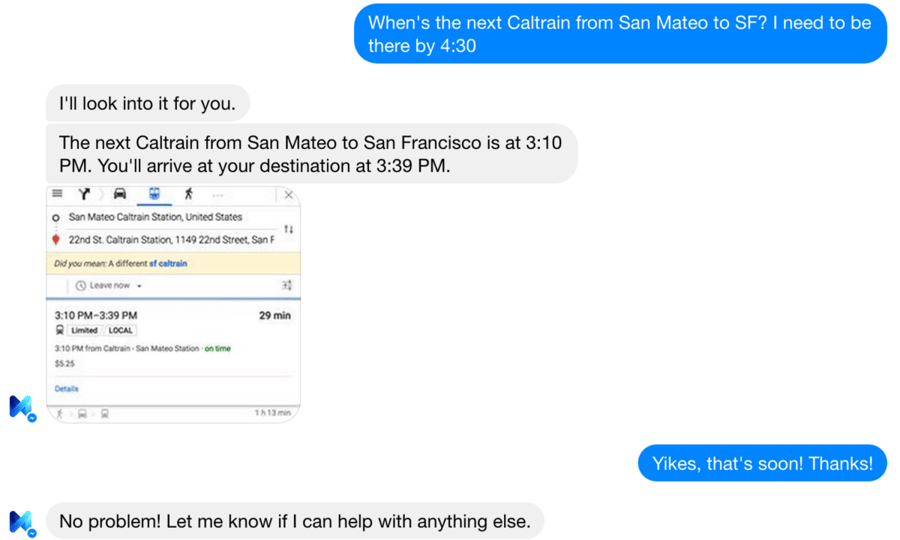Screenshot of a Chat Interaction: Planning a Caltrain Trip from San Mateo to San Francisco

In this well-detailed screenshot, a conversation between a user and what appears to be an AI assistant unfolds. The user inquires, "When's the next Caltrain from San Mateo to San Francisco? I need to be there by 4:30." The AI assistant responds, stating, "I'll look into it for you."

The AI then provides specific details: "The next Caltrain from San Mateo to San Francisco is at 3:10 PM. You'll arrive at your destination at 3:39 PM." Accompanying this message is a screenshot of a website that displays the route information: San Mateo Caltrain Station to 22nd Street Caltrain Station, located at 1149 22nd Street, San Francisco. Additionally, the website queries, "Did you mean a different Caltrain?"—underscoring the AI's attempt to ensure accuracy.

The AI reinforces the timing, "3:10 PM to 3:39 PM, a 29-minute journey," with a further detail about the fare: "$5.25 for the trip." The user, seemingly surprised by the imminent departure, responds, "Yikes, that's soon. Thanks." The AI replies reassuringly, "No problem, let me know if I can help with anything else," ending the conversation on a helpful note.

Through this interaction, the meticulous sequence and the efficient resolution detail the AI's capability in assisting with public transportation inquiries, all while maintaining a polite and supportive tone.